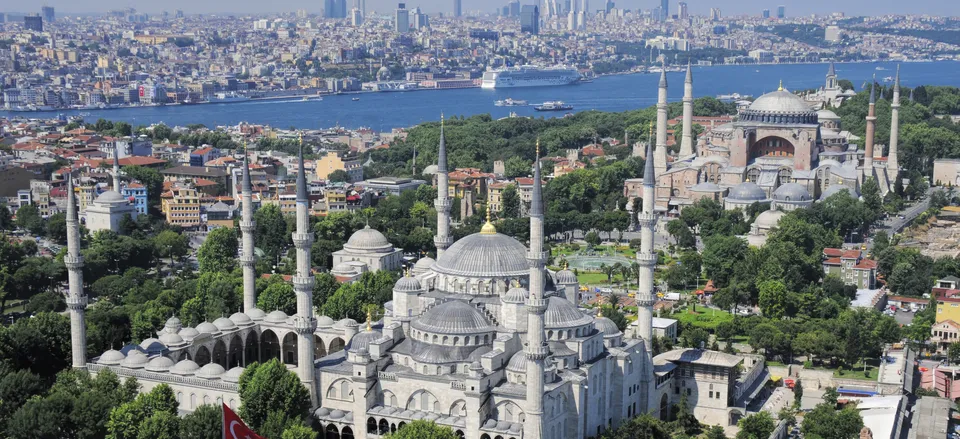This is an aerial photograph of a large, bustling city divided by a prominent river running horizontally across the middle of the image. Dominating the foreground are two impressive mosque-like buildings with multiple domes and tall, pointed steeples. One mosque appears primarily white with a distinctive dome featuring a yellow tip. In contrast, the other mosque exhibits darker colors. The area surrounding these temples is lush with green trees, speckled with smaller buildings and possibly a fountain or small pond nestled between the two mosques.

Further back, on the opposite side of the river, the city continues with a mixture of houses, mid-sized buildings, and a few towering skyscrapers. A large cruise ship is docked on the riverbank, accompanied by several smaller boats navigating the waters. The photograph is taken during the day, providing a clear view of the intricate details of the city's architecture and landscape. However, there are no visible signs indicating the specific location or country of this striking cityscape.